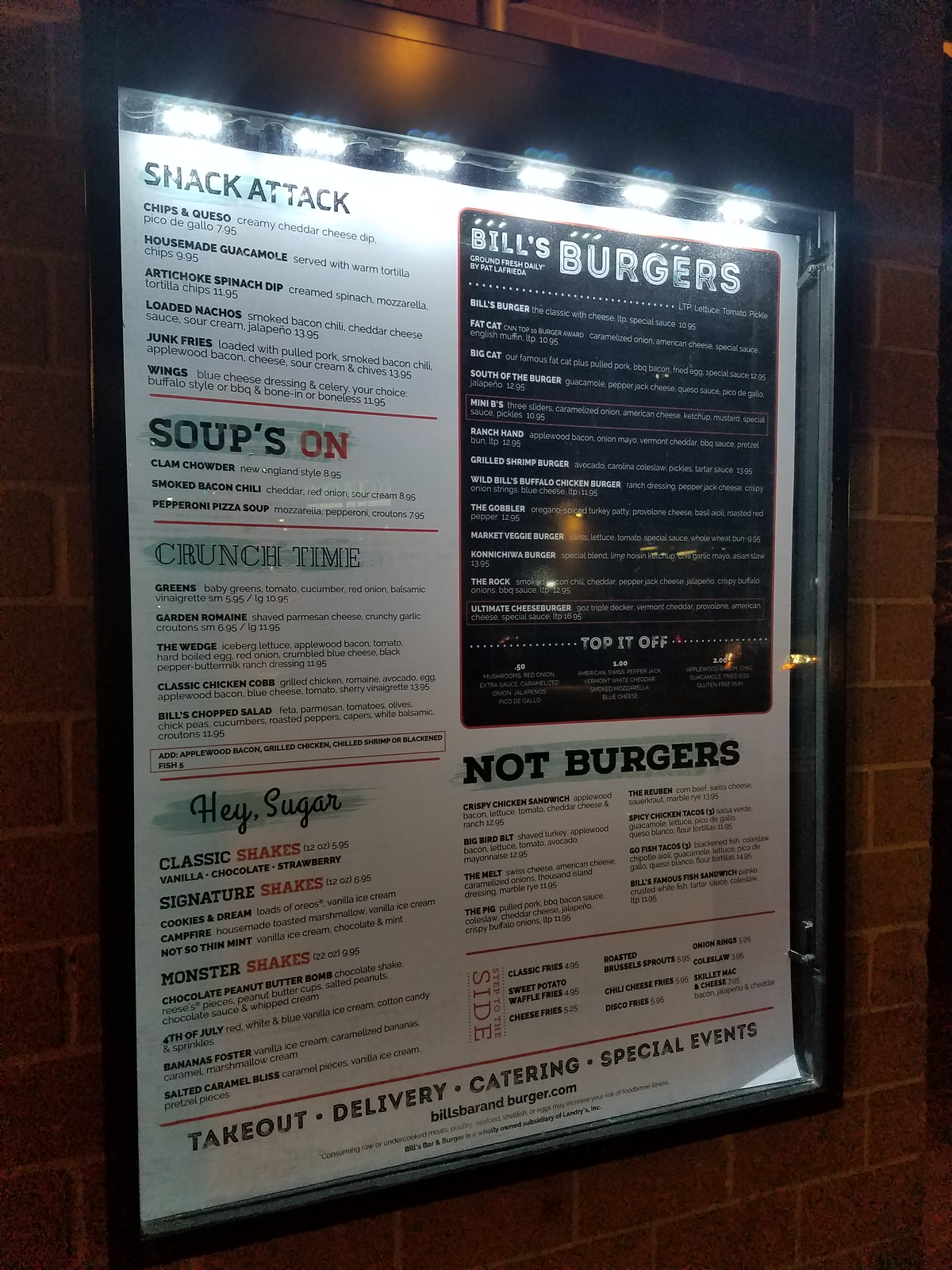The digital photo, taken outdoors later at night, features a tan brick wall with white mortar between the bricks, framing the entire scene. Dominating the image is a black box mounted on the wall, containing a large, laminated white menu behind a glass front. At the top of the box, six small, brightly lit LED lights illuminate the menu, and a silver rod at the top center appears to house the electrical components.

The white menu inside the box displays several sections in different fonts and colors. In the upper left corner, the words "Snack Attack" are prominently written in bold black text. Adjacent to this, the phrase "Suits On" is highlighted with green over black text. Below it, "Crunch Time" appears in bubble lettering, featuring black edges and white interiors accented with green highlights. The phrase "Hey Sugar" is elegantly penned in a lighter black cursive font, also highlighted in green.

In the top right corner, a prominent black square with white text reads "Bill's Burgers" and lists various burger options. Below this, another section titled "Not Burgers" is highlighted in green over black text. The bottom of the menu emphasizes important details in bold text, stating "Takeout, Delivery, Catering, Special Events," and provides the website Bill'sBarredBurger.com.